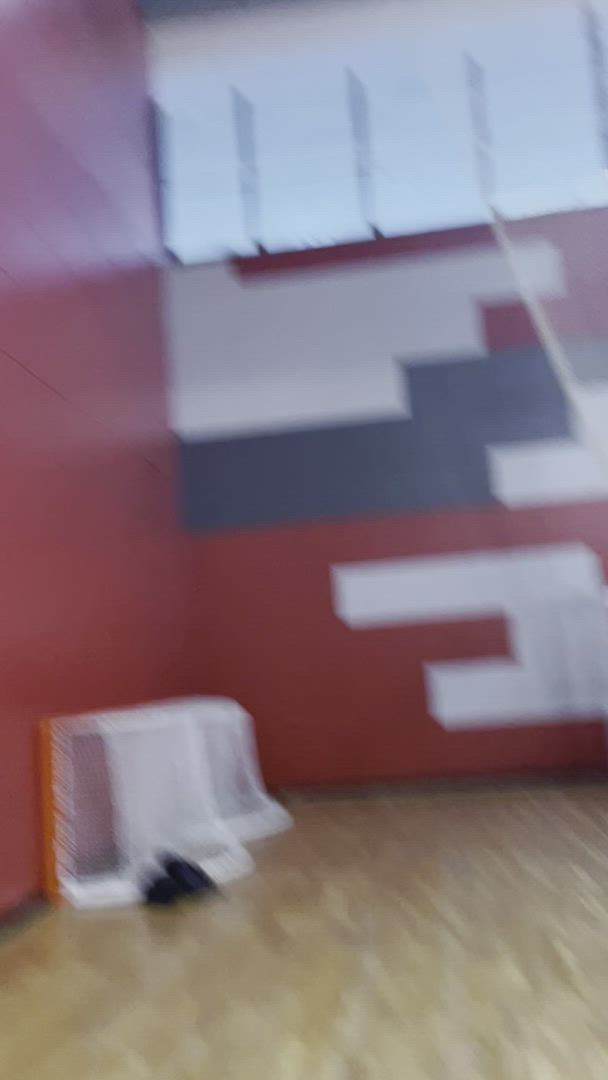A very blurry photograph captures a room with bold red walls. The dominant feature on the left side is a diagonally slanted red wall, extending towards a corner where it transitions into a horizontal wall along the top part of the image. The lower right portion of the red background wall showcases a white geometric design, while above it, a pattern of dark blue or black mixed with additional white geometric elements emerges. In the upper right corner, at the top edge of the red wall, a series of four very bright windows cast a luminous white glow. The flooring is indistinct due to the blur, appearing to be either wood or tan carpet. Near the left corner, where the side wall meets the back wall, two small, conical white objects can be seen, their shapes too indistinct to identify clearly.